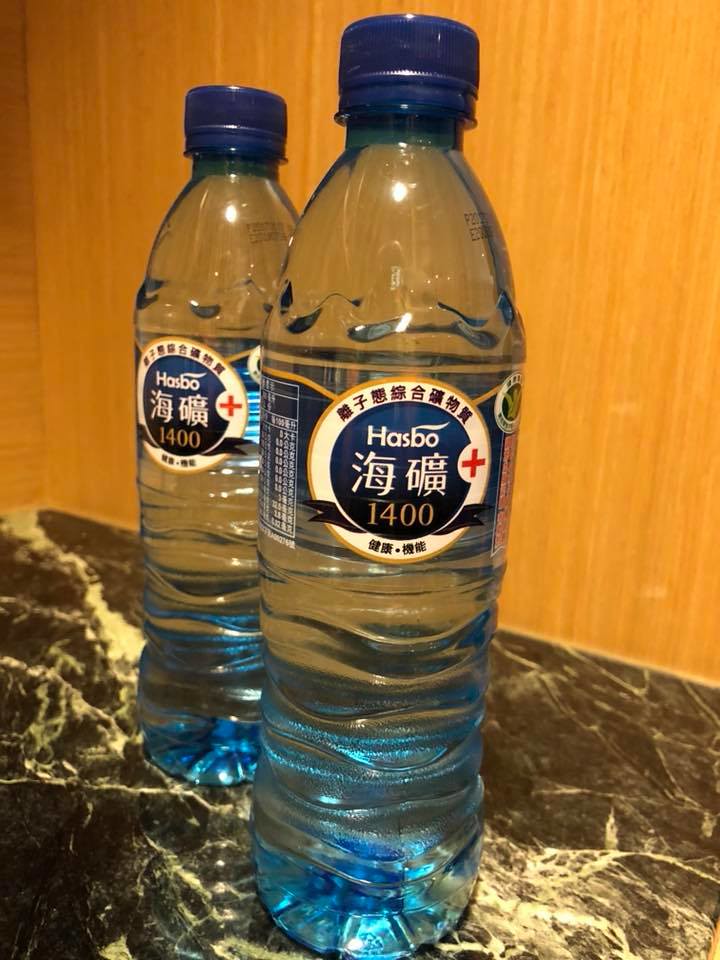This is a detailed photograph of two translucent blue water bottles with dark blue caps, positioned on a black and white marble countertop. One bottle stands prominently in the center, while the other is slightly to the left and behind it. The primary label on the bottles features a blue circle encircled by white and a thin gold trim. Within the blue circle, the brand name "Hasbo" is displayed in stylized text, followed by two significant kanji characters, and the number "1400" beneath them. Surrounding this central portion, additional kanji characters are printed at the top and bottom of the white circle, with a red plus sign nestled on the right side of the logo. The background of the image showcases a panel of light oak-colored wooden veneer, enhancing the overall aesthetic.